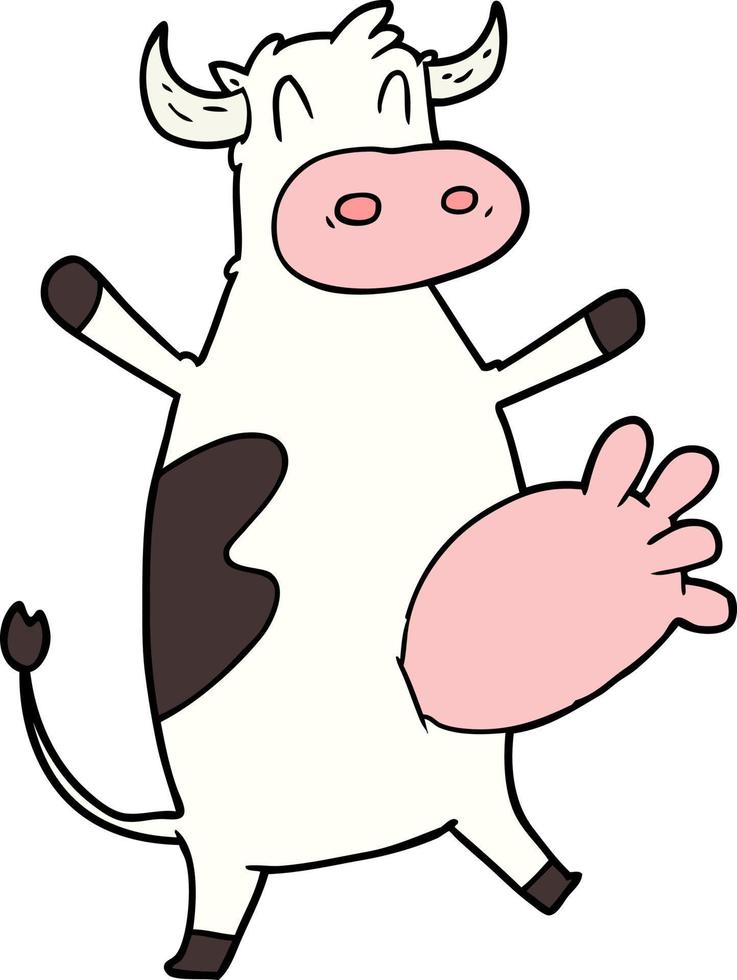This is a cartoonish clipart-style image of a dairy cow standing upright on its hind legs, facing the viewer with outstretched front legs. The cow's body is predominantly white with a notable black splotch on its left side, and it has a distinctive curled white tail tipped with black. Its legs are white, ending in black-tipped hooves. The cow's capsule-shaped pink nose features two darker pink circles for nostrils. The eyes are depicted as two black, upside-down U-shaped curves, emanating a cheerful expression without a visible mouth. The cow sports slight gray horns outlined in black. Rising next to its body is an unusually large pink udder with four nipples, almost balloon-like in its exaggerated form. The image also shows some small details like hair on top of the cow's head, enhancing its playful, whimsical appearance.